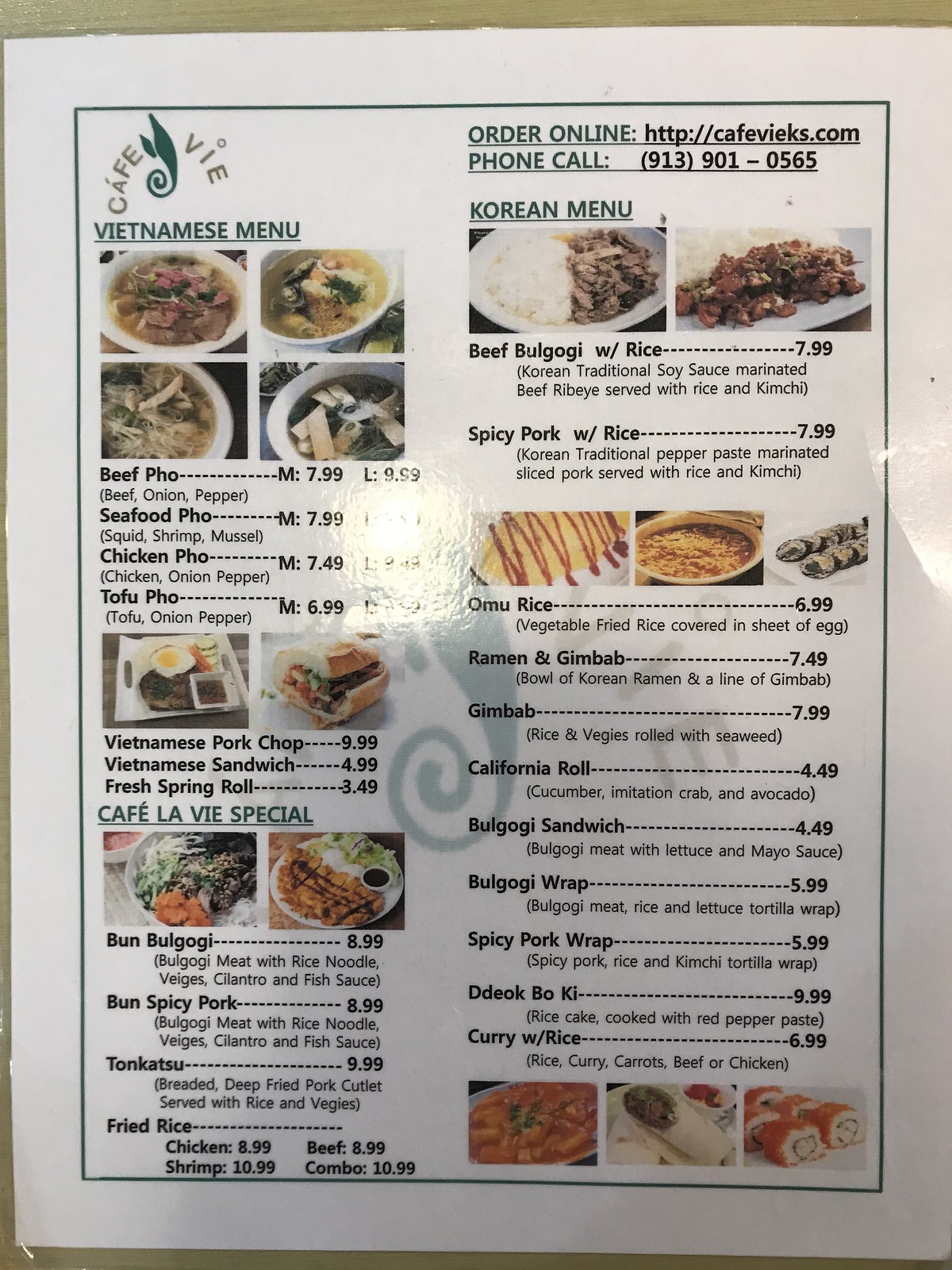This detailed description presents a photo of a laminated, glossy menu from Cafe Vie. The menu rests on a light brown, potentially wooden table, visible near the top and bottom edges.

**Top Section:**
- **Top Left Corner:** Displays the "Cafe Vie" logo in light gray letters accompanied by a dark green symbol.
- **Under the Logo:** The title "VIETNAMESE MENU" appears in all capital, sans-serif letters, underlined.
- **Beneath the Title:** Four rectangular images of soups in white bowls.

**Middle Section:**
1. **Beef Pho:** 
   - Price: $7.99 (medium), $9.99 (large).
   - Description: In parentheses, it says "beef, onions, and peppers."
2. **Vietnamese Pork Chop:**
   - Price: $9.99.
   - Image: Plate meal.
3. **Vietnamese Sandwich:**
   - Price: $4.99.
   - Image: Small sandwich.
4. **Fresh Spring Roll:**
   - Price: $3.49.

**Special Section:**
- **Title:** “CAFE VIE SPECIAL” in larger, all-capital, green letters.
- **Images:** Two side-by-side colored images of unspecified dishes.
1. **Fun Bulgogi:**
   - Price: $8.99.

**Right Column:**
- **Title:** “ORDER ONLINE” (http://cafevieks.com)
- **Phone:** (913) 901-0565 (both in black letters).
- **Section Title:** “KOREAN MENU” underlined in green letters.
- **Images:** Two images of Korean dishes.
1. **Beef Bulgogi with Rice:**
   - Price: $7.99.
   - Description: “Korean traditional soy sauce marinated beef ribeye served with rice and kimchi.”
2. **Additional Items:**
    - More items listed with images, including another description and a list of ten more menu items with corresponding images towards the bottom.

This caption aims to provide a detailed visual and text-based description of the Cafe Vie menu, ensuring the layout and chronicling distinct elements presented in the photograph.